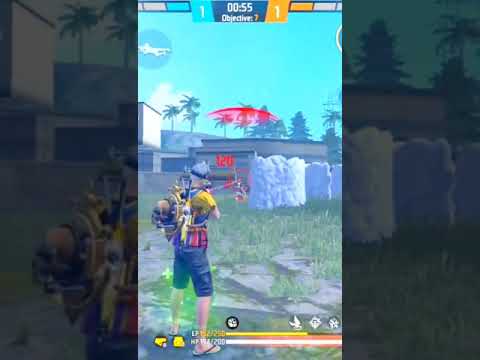This image is a detailed screenshot from a colorful video game, likely depicting an action scene. In the background, palm trees and a hill with pine trees are visible against a light blue sky, flanked by broken pillars and various rectangular, brown and gray buildings. The photograph, seemingly captured on a vertical camera phone, shows a man, the in-game character, positioned off-center to the left. He is facing away from the camera, shooting something with a weapon emitting red effects. He sports short silver or gray hair, a yellow shirt, dark knee-length shorts, black sandals, and a black backpack filled with various items, including a notable skull emblem. His calves are exposed, and his attire includes goggles on his head.

Prominently displayed on the screen are game HUD elements: at the bottom, yellow and white bars indicate health and objective status, showing 00:55 seconds and Objective 7. The top center of the screen highlights a score of 1-1 between a teal square on the left and an orange square on the right. Additional elements include meters on both the top and bottom, likely showing player stats and a score indicator reading "125" in red. The entire scene is captured from a third-person perspective, with detailed in-game graphics emphasizing the dynamic environment and the character's equipment.